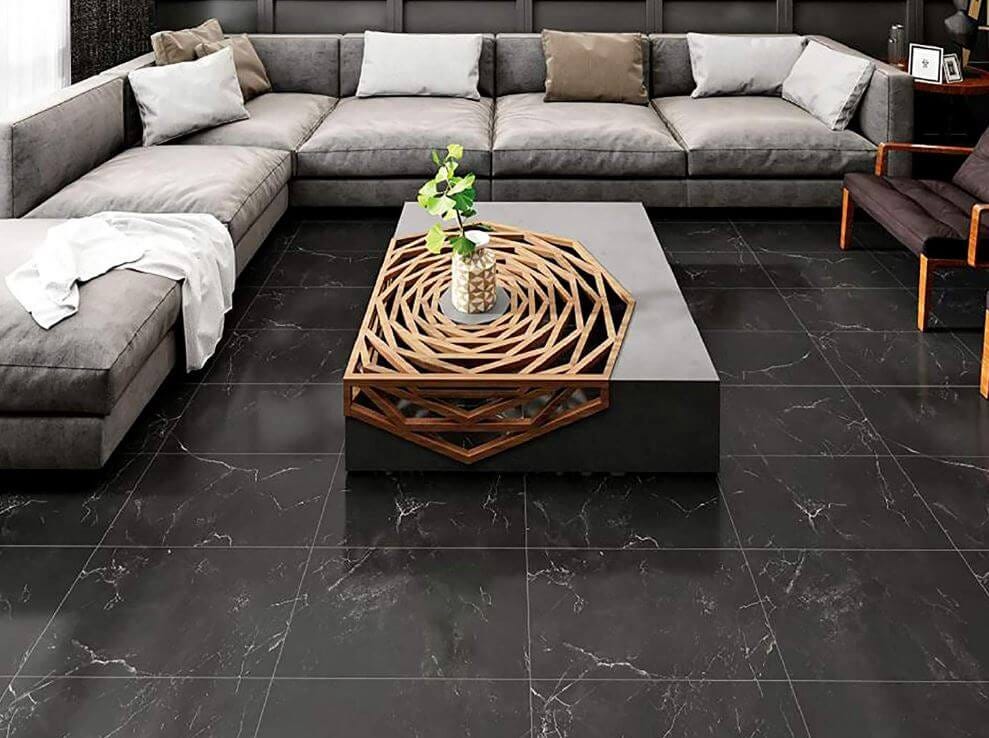The image captures an elegantly staged living room, perfect for an interior design magazine. The floor features dark marble tiles with striking white veining. Dominating the left and back sides is a low-to-the-ground, beige sectional couch with wide, large cushions and a short back, making it appear inviting and comfortable. Scattered across the couch are throw pillows in shades of cream and dark brown, accompanied by a small, cream-colored blanket draped over the right-hand side.

The centerpiece of the room is a unique and intriguing coffee table. This table is a solid block of gray material, positioned low to the ground. What truly sets it apart is the geometric cutout section on the closest left-hand side. This cutout features a hexagon-shaped design made of light-colored wood, creating a stunning spiral pattern that extends from the top of the table down to the side, blending seamlessly into the lower half. At the center of this wooden design sits a white and brown vase housing a vibrant green plant, adding a touch of nature to the sophisticated setting. 

In the right part of the image, a chair with a black cushion and wooden brown frame complements the overall decor. The room's polished aesthetic, filled with carefully chosen elements, makes it an exemplar of refined interior design.